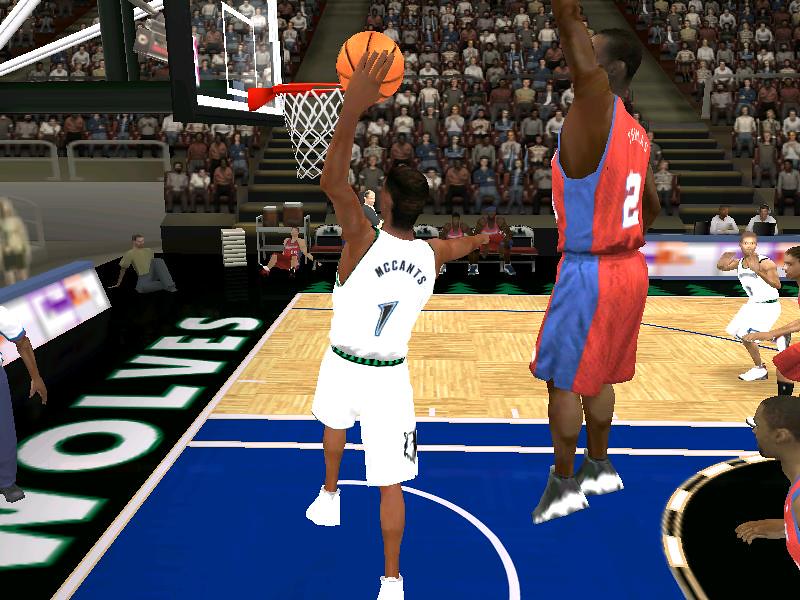This image, a screenshot from a video game with graphics reminiscent of the Xbox 360 and PS3 era, captures an intense moment in a basketball game featuring the Timberwolves. The scene centers on a player in a white jersey with a green waistband, identified as number one, McCants. He is airborne, ball in his left hand, poised to dunk. Beside him, a player in a blue, white, and red jersey leaps in a likely futile attempt to block the shot, as he's positioned slightly behind McCants. The floor beneath and behind the hoop is painted blue, displaying the word "Wolves" in white text. In the background, the court features light wood with blue and black accents, including a prominent black circle. Additional players from both teams are visible running towards the action. The audience, filling every seat, remains static, hinting at the game being in a non-playable state or paused. To the right, the players' bench can be seen with some team members waiting to substitute. The overall impression suggests an exhilarating moment in a digital depiction of this basketball showdown.